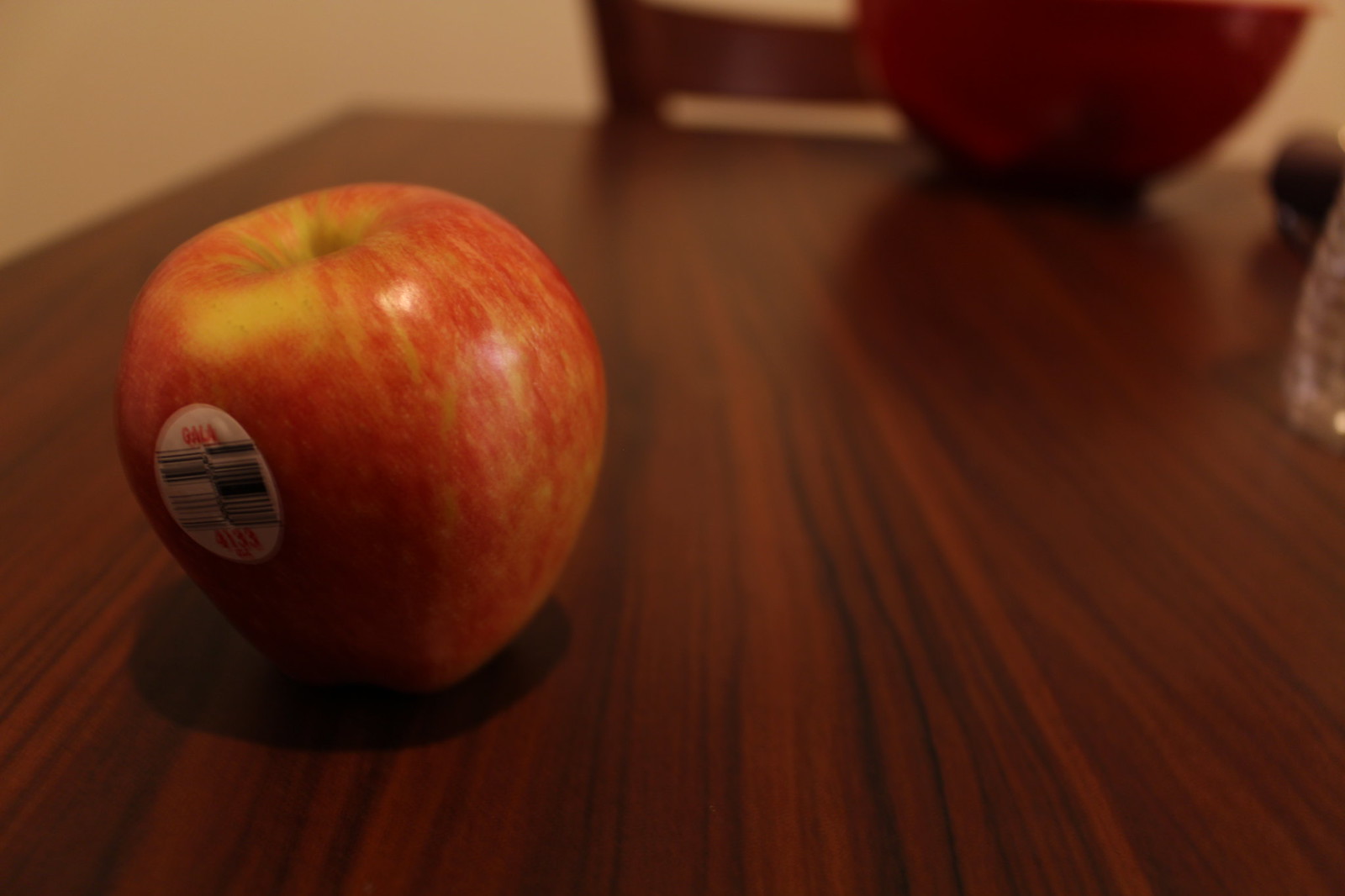The image depicts a blurry close-up of a dining room table surface, allowing for detailed observation of the table's wood grain. The wood grain appears almost too perfect, giving the impression of a veneer on top of fake wood. In the foreground, to the left, stands a mostly red apple with a few green specks. The apple is upright and bears a white oval sticker from the grocery store, labeled "Gala" in red font, along with a barcode and the number 4133 in red.

To the right side of the image, the bottom of a water bottle is visible, with an indiscernible small black object behind it. In the upper right corner, part of a fruit bowl can be seen, indicating the table is used for dining. Just behind the fruit bowl, the tip of a chair is noticeable, suggesting a chair is pushed in at the table. Despite the overall blurriness, the wooden table's surface details stand out prominently.